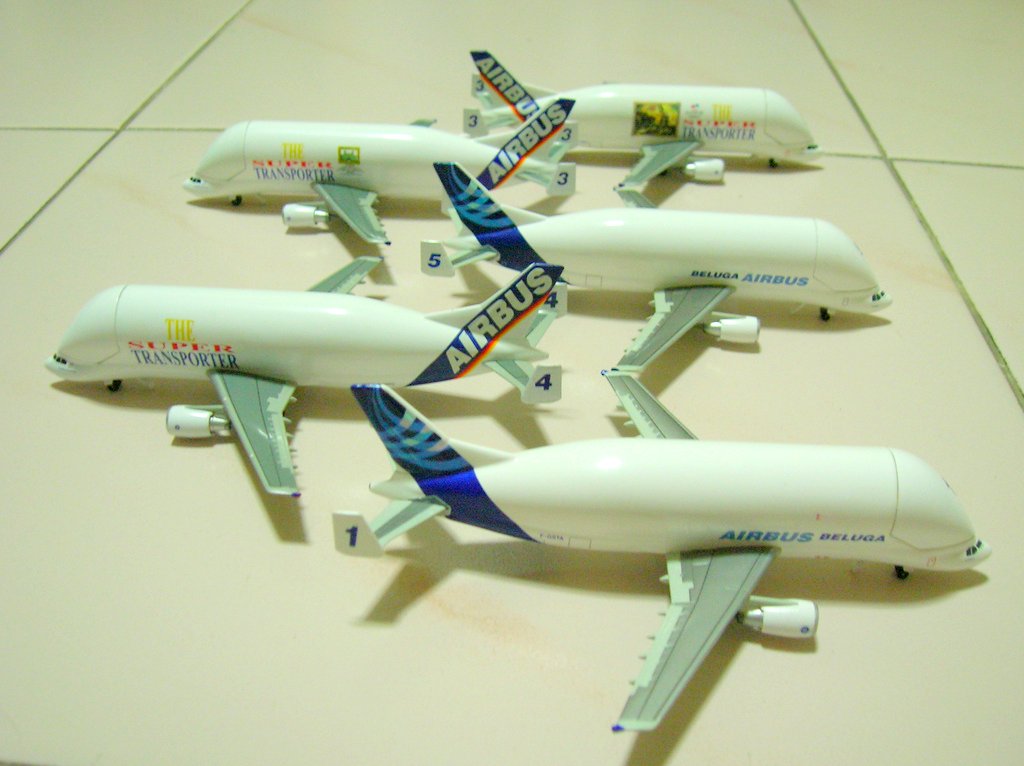The photograph is a dimly lit, amateur shot of five model planes arranged on a floor made of large ceramic tiles, evident from the visible grout, which is dark grey with lighter, uneven tones. The models, representing Airbus transport cargo planes, have a distinctive wide body and are white with red and blue wording. The planes are identifiable as Airbus Belugas and Super Transporters, each marked with the Airbus logo on their blue tails. The planes' positioning is methodical; starting from the forefront, they alternate directions, with the first facing right, then left, and so on. Their arrangement runs down the center of the image with all tails aligned centrally. Each model is numbered from one to five, though the specific order is not clear. The cockpit area of these planes features a notable cutout design at the nose for loading large cargo. Despite the photo's lack of sharp focus, these details are distinguishable, giving the impression of an enthusiast's collection displayed on a kitchen-like tile floor.